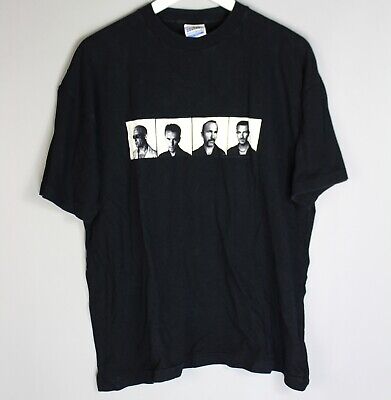This image features a short-sleeved black cotton t-shirt displayed against a light gray background, resembling a product photo typically seen on retail websites. The shirt is hanging on a white coat hanger, with a small, unreadable tag visible at the back of the neck. The fabric appears wrinkly, suggesting it could either be pre-owned or designed in a vintage style. Centered on the t-shirt's chest is a graphic comprised of four small, square, black-and-white photographs. These photos depict four men, likely the band members of U2. Three of the men wear dark shirts, while the man on the left dons a white shirt and glasses. All the men appear to have brown hair, with two sporting mustaches. The surrounding background of each square photo is white, enhancing the contrast against the black t-shirt.